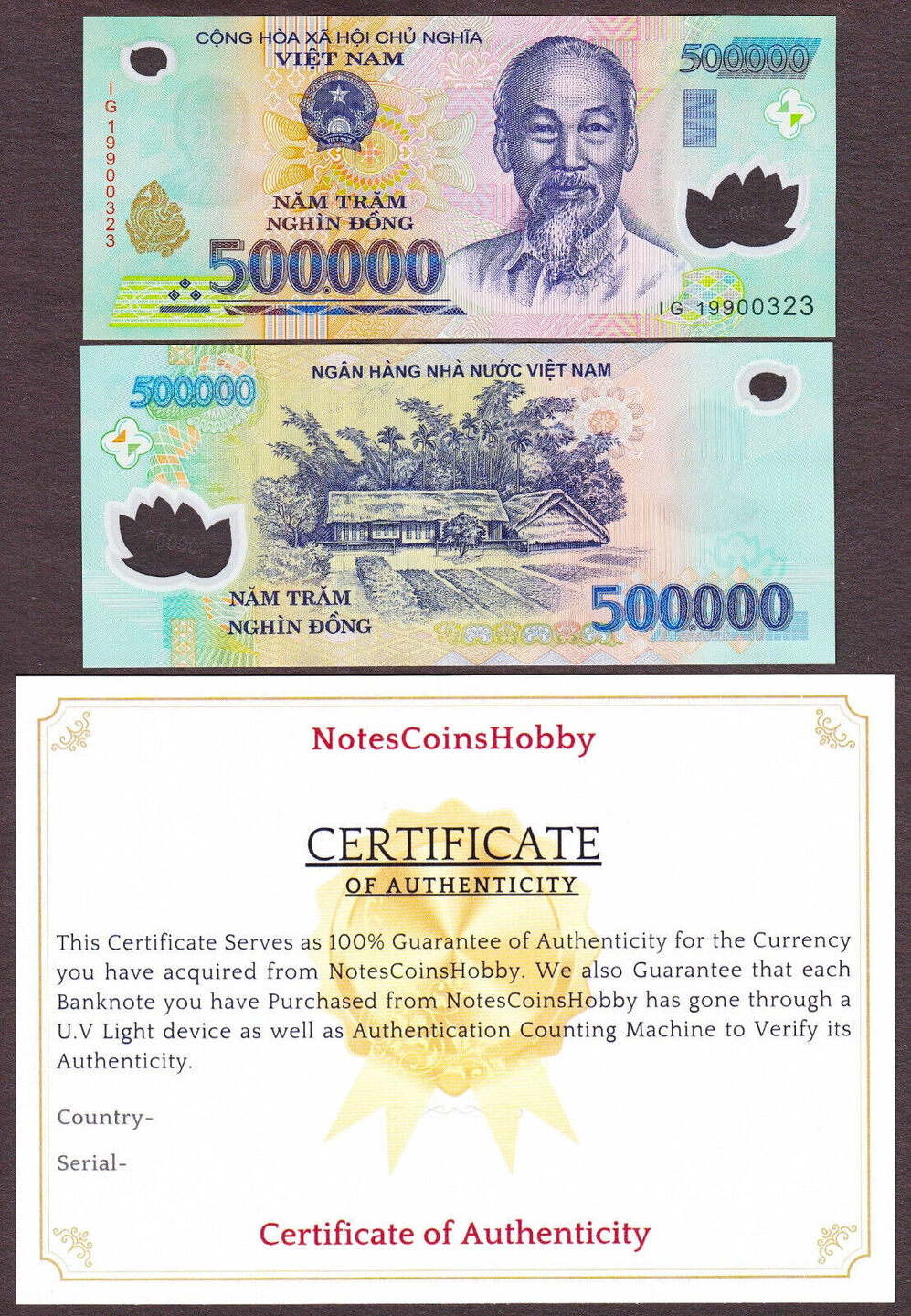The image showcases Vietnamese currency, depicting both the front and back sides. The front of the banknote features a portrait of a distinguished Vietnamese man with a white beard, likely a significant historical figure, set against a colorful backdrop of teal, blue, and yellow hues. The top right corner indicates the denomination of 500,000. The reverse side of the note displays a small rectangular house surrounded by trees, all rendered in a more subdued black-and-white palette. Adjacent to these images, the image includes a white certificate of authenticity, adorned with golden lettering and designs. This certificate, issued by Notes Coin Hobby, guarantees the authenticity of the currency. It includes a prominent golden ribbon and details the verification process through UV light devices and authentication counting machines, ensuring the genuineness of the banknotes.